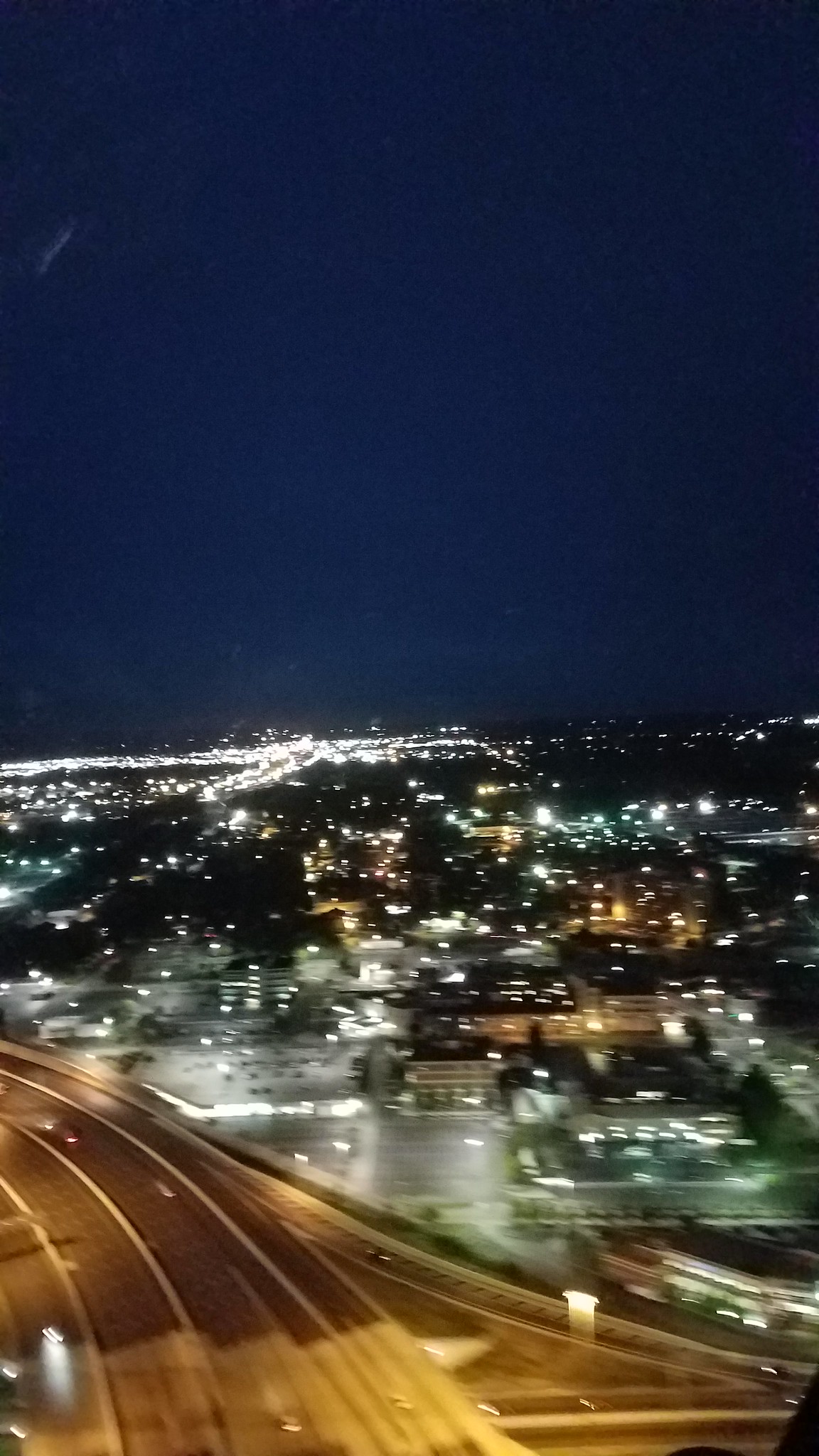This image, while quite low in quality and resolution, captures an outdoor scene from an aerial perspective. The top portion of the image displays a predominantly dark blue sky. On the bottom left, there are roads intersecting and branching off in multiple directions, with several indistinct cars visible on them. The blurriness makes it difficult to determine the exact number of vehicles. In the background, the faint outlines of buildings can be seen, indicating an urban area.